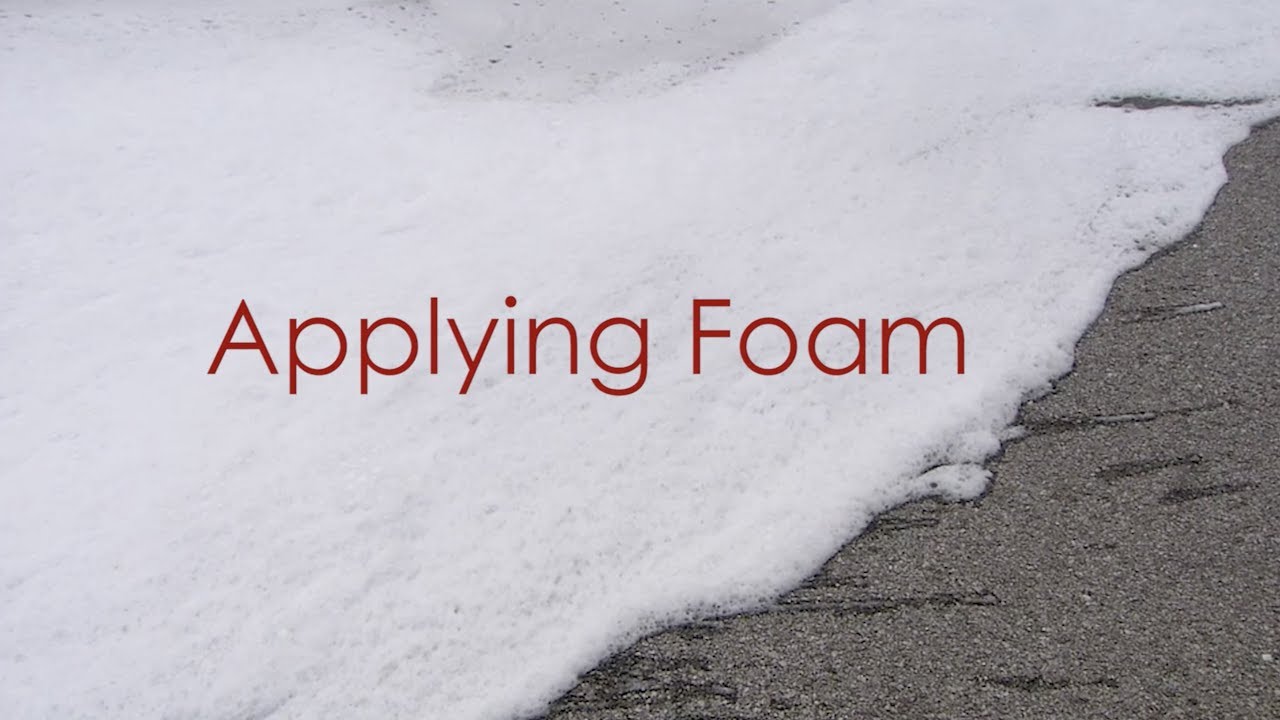This is a realistic photo depicting an older, sun-faded asphalt surface covered almost entirely by a white, foamy substance, resembling a cleaning agent or preparation foam. The image captures the textured contrast between the rough, lighter gray asphalt visible on the right edge and the dense white foam that blankets approximately 80% of the surface. Prominently displayed in the middle of the foam in deep red letters is the text "applying foam," suggesting a cleaning or preparation process. The font appears to be either Verdana or Times New Roman. The overall impression is that the image could be an online stock photo meant for tutorial or instructional use.